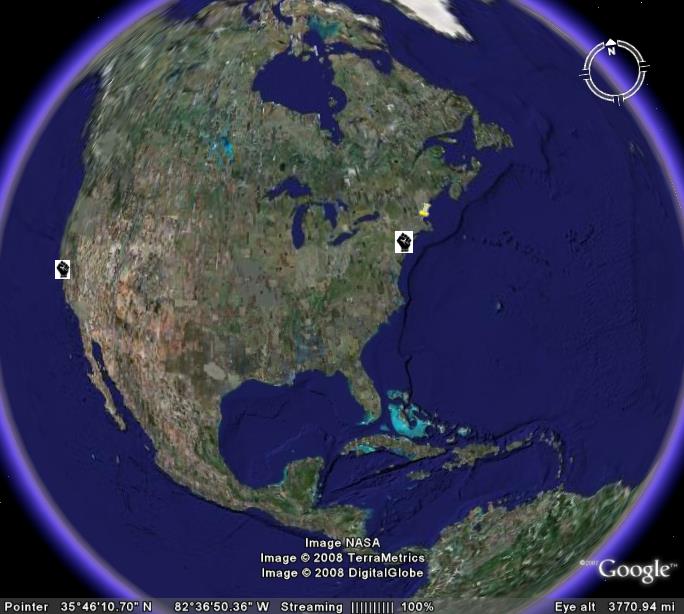This detailed image is a screenshot from an earlier version of Google Earth, specifically the 2008 edition. It showcases a digital and somewhat inaccurate depiction of the North American continent, stretching from the upper reaches of Canada covered in white snow to parts of Central America, the Caribbean, and the tip of South America where Brazil would be located. The primary colors on the map are green shades for most of the U.S., Canada, parts of Mexico, and South America, while the arid regions in the southwest are depicted in dusty hues.

Prominently displayed are two highlighted locations: New York City, New York, and near San Francisco, California. The image is wrapped around a globe, mimicking a view from space with oceans depicted in deep blue bordered by a purple ring, and black fading into the edges. 

Text on the map includes "2008," with credits to "Terrametrics" and "Digital Globe," and it appears to be streaming at "100%." Coordinates mentioned in the image are 35 degrees 46.10.70 N, 82.36, 50.36 W, though this exact point is difficult to identify on the map. Additionally, it features a logo that resembles a hand grasping with thumbs and fingers tucked in, next to a compass pointing north in the top right corner, adding more layers to the map's intricate details.